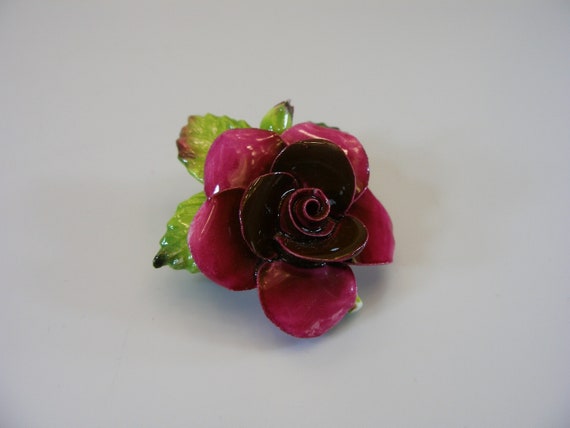The image is a detailed photograph of a handcrafted glass rose resting on a light gray surface. The rose features a dark purple center followed by three dark red inner petals, transitioning to five dark pink outer petals. Accentuating the flower are a few semi-transparent light green leaves. The glass has a shiny, reflective quality, enhanced by a light source positioned above, casting a shadow below the flower. The intricate details and shimmering texture of the glass emphasize its artistry, possibly categorizing it as a piece of fine art or jewellery.